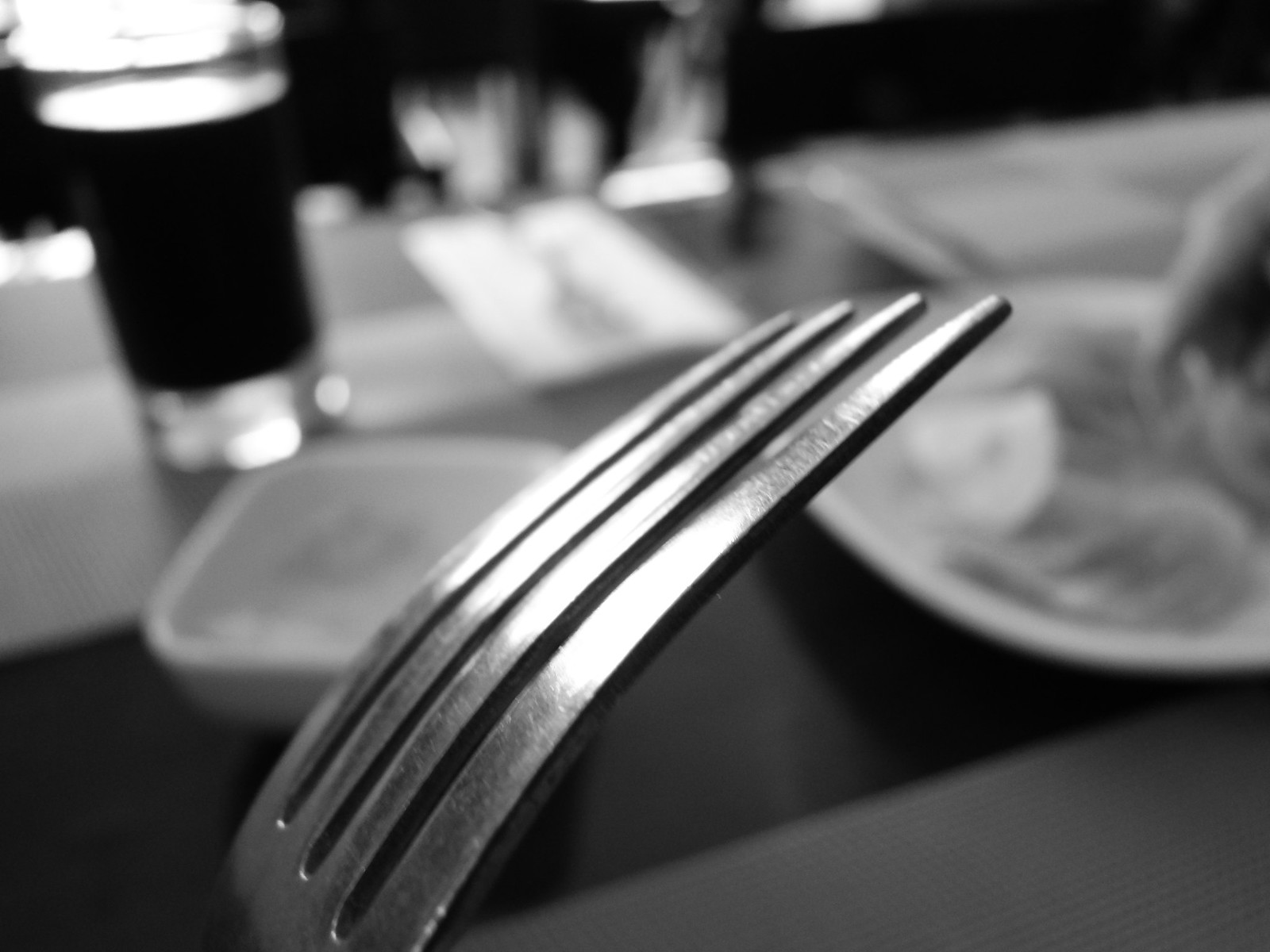This black and white close-up photograph prominently features the four prongs of a silver fork, occupying approximately 75% of the image's height and 40-50% of its width. The fork is so near that its handle is not visible, creating a sharp contrast with the blurred background. Behind the fork, to the left, lies a square white saucer or plastic tray, which seems empty. Further in the background, slightly out of focus, there is a dinner table setup with various items. 

A glass cup, filled nearly to the top with a dark liquid similar to cola, is noticeable due to its bright surface reflection. To the right of the fork, there is a large, blurred plate that possibly contains indistinct food items, such as a filleted meat or dinner roll. There is also a white napkin with another fork resting on it next to the plate. The background objects are partially obscured, adding a sense of depth to the image. The table itself, which appears checkered in pattern, might be covered with a white cloth. Together, these elements suggest a casual dining scene, possibly in a restaurant setting.